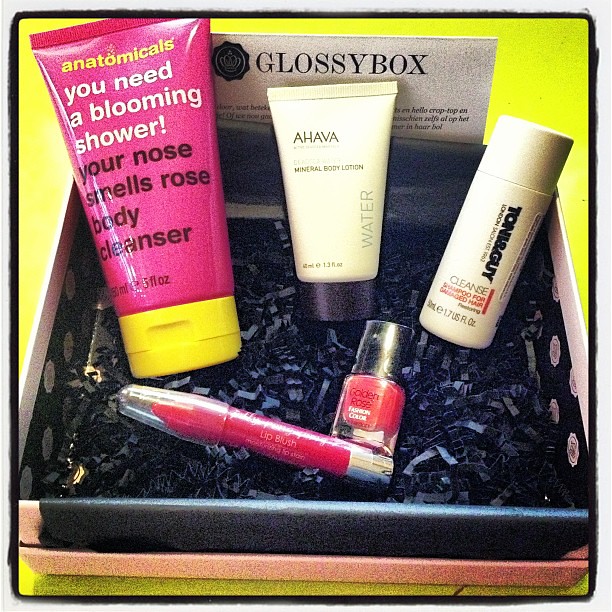In the image, a neatly arranged white box filled with various personal care products is displayed against a lime green background. The box, adorned with black confetti at the bottom, is identified by a card that reads "Glossy Box" in bold black letters. Inside, the most prominent item is a vibrant pink tube with a yellow cap, labeled "anatomicals you need a blooming shower, your nose smells rose body cleanser." Next to it is a white tube of Ahava mineral body lotion, slightly smaller but with a similar shape. There's also a small white bottle with black lettering, likely a cleansing shampoo for damaged hair. Among the items, there are a pinkish-orange nail polish sample and a dark pink, chubby lip liner placed horizontally at the bottom of the box. Additionally, there are small containers of lip blush and lip gloss, contributing to the colorful and visually appealing assortment of products.